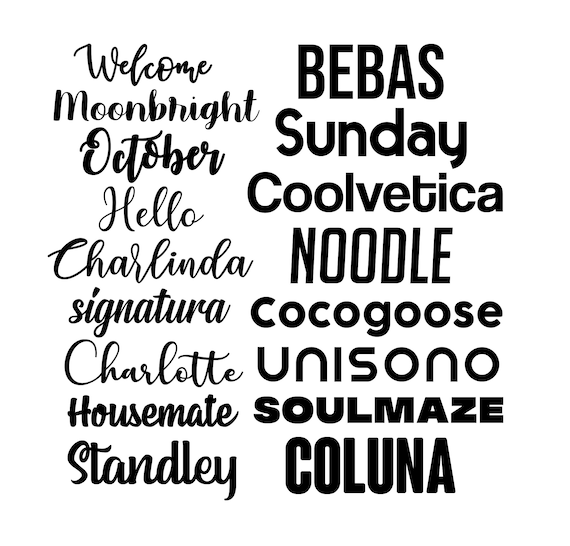The image displays a white background with a simple black ink. It features a series of words organized in two vertical columns. The left column showcases stylized fonts with words such as "Welcome," "Moon Bright," "October," "Charlinda," and "Charlotte." Contrastingly, the right column lists these words again but in a simpler serif or sans-serif font style, appearing as labels or names for the fonts used in the left column. For instance, "Welcome" in a more decorative font is matched with "Bebas" on the right, "Moon Bright" with "Sunday," "October" with "Coverica," and "Charlinda" with "Kaluna." The systematic pairing suggests that the left side provides an example of each font's appearance while the right side names each font. Overall, it presents twelve pairs of words, each pair illustrating the same word in two distinct typefaces against a minimalistic white backdrop.